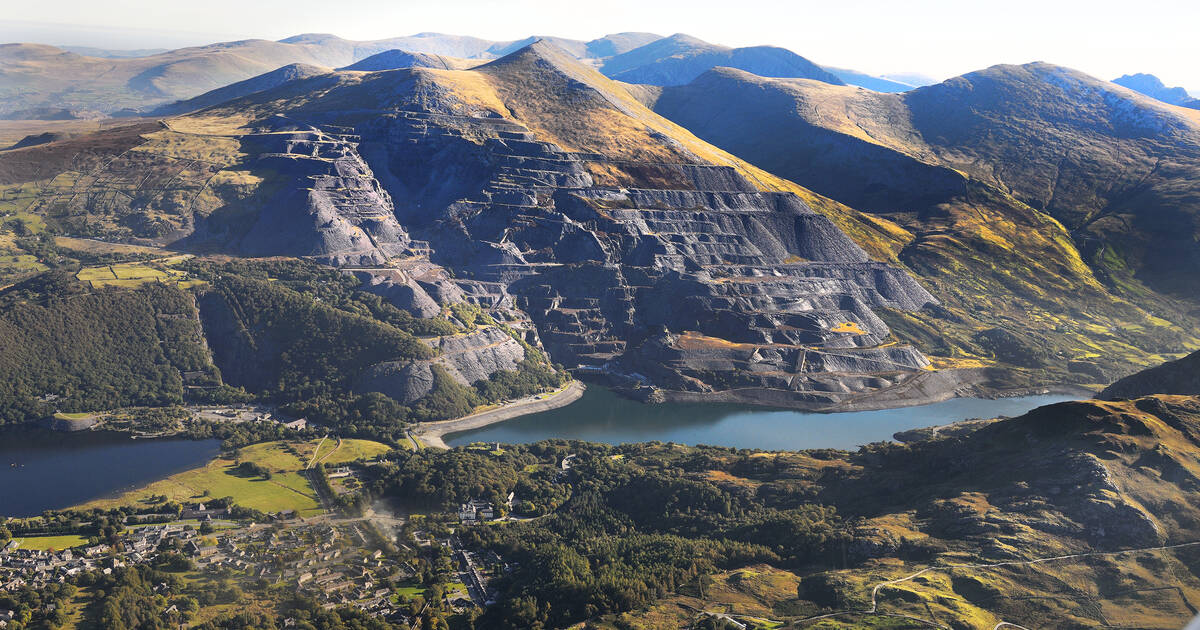The image presents a striking outdoor view of a vast mountain range illuminated by the sun, creating a hazy white sky backdrop. In the center of the image, a river meanders through the verdant valley, flowing from the bottom left towards the middle right. The mountains are covered with lush greenery, ranging from light to dark green, highlighting the rich vegetation. Notably, some mountainsides feature tiered formations, resembling steps, which could be natural or human-made, possibly hinting at strip mining activities. At the bottom left, a small rural village nestles among the rolling hills and trees, partially obscured and distant. The rocky terrain, interspersed with green trees and grass, adds to the intricate landscape, showcasing a blend of natural beauty and subtle human impact.